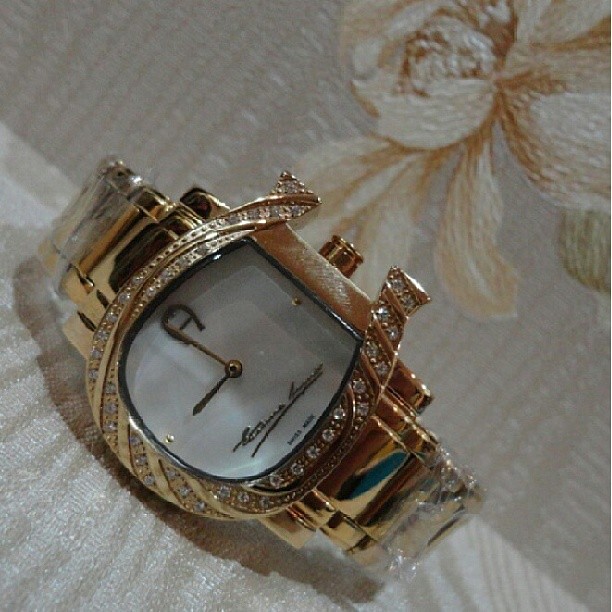This image features a uniquely designed gold watch with a distinctive C-shaped frame. Viewed from different angles, the frame resembles a golden horseshoe outlined with sparkling diamonds. The entire structure, including the watch's casing and wristband, is crafted from luxurious gold. The face of the watch is a crisp white, notably without any numerical markers. Instead, a gold dot marks the three o'clock and nine o'clock positions. At the bottom of the watch face, the designer's name is inscribed in cursive, though it appears somewhat illegible. The combination of gold and diamonds, along with the clean white face, gives this timepiece an elegant and sophisticated appearance.